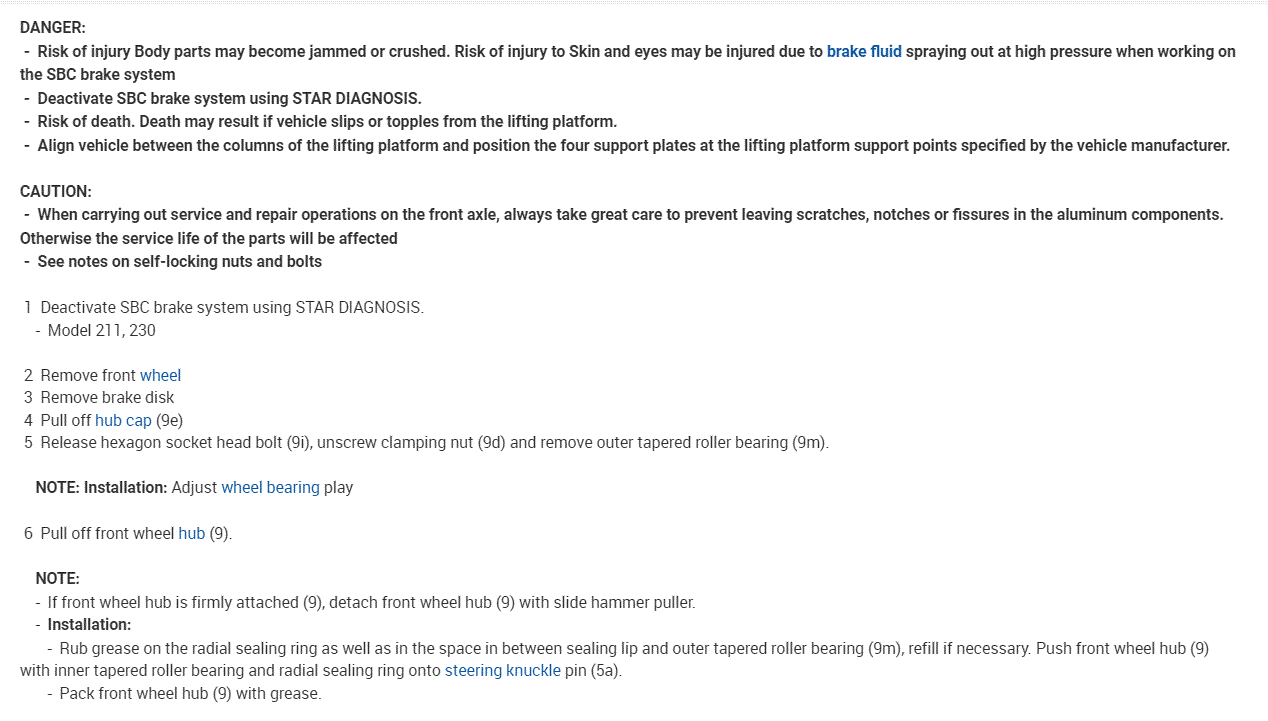**Detailed Caption:**

The image is composed solely of text on a plain white background. At the very top, in prominent black lettering, the word "Danger" is highlighted. Beneath this, a detailed warning is provided: 

"Risk of injury. Body parts may become jammed or crushed. Risk of injury to skin and eyes may occur from brake fluid spraying out under high pressure when working on the SBC brake system." Notably, the term "brake fluid" is emphasized in blue text.

Following this, an advisory in bold letters states: "Deactivate SBC brake system using star diagnosis."

A severe warning is then displayed: "Risk of death. Death may result if vehicle slips or topples from the lifting platform." 

Guidelines on vehicle placement follow: "Align the vehicle between the columns of the lifting platform and position the four support plates at the lifting platform. Support points as specified by the vehicle manufacturer."

A cautionary section underscores the importance of careful handling during service and repair: 

"When carrying out service and repair operations on the front side, always take care to prevent leaving scratches, notches, or fissures in the aluminum components. Otherwise, the service life of the parts will be affected. See notes on self-locking nuts and bolts."

The text then transitions into a step-by-step procedure for handling brakes, enumerated from one to six:

1. Deactivate SBC brake system.
2. Remove the front wheel.
3. Remove the brake disc.
4. Pull off the hub cap.
5. Release the hexagon socket head bolt.
   
A note specifies post-installation instructions: "Adjust wheel bearings play."

Finally, number six in the list states: "Pull off the front wheel hub."

This comprehensive set of instructions seems to provide essential safety warnings and a detailed procedural guide for dealing with the SBC brake system, aimed at preventing injury and ensuring proper maintenance.